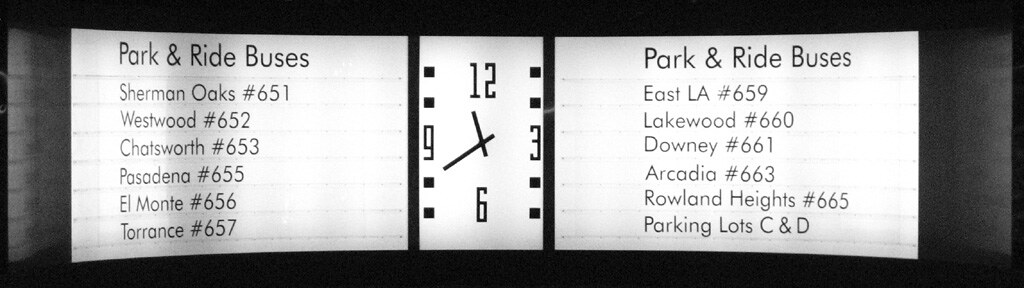The image displays a digitally created bus depot sign, characterized by its clean, almost video game-like appearance, which renders it somewhat unrealistic. The sign is split into two sections with "Park and Ride Buses" headers on both the left and right sides, each listing different destinations. On the left, it lists Sherman Oaks (651), Westwood (652), Chatsworth (653), Pasadena (655), El Monte (656), and Torrance (657). On the right, it enumerates East LA (659), Lakewood (660), Downey (661), Arcadia (663), Roland Heights (665), followed by Parking Lots C and D. Centered between these sections is a white rectangular clock face with black markings, displaying only the numbers 12, 3, 6, and 9, and dots in place of the other hour markers. The clock reads approximately 11:43. The overall background of the sign is black, contrasting with the white sections where the text and clock are displayed.